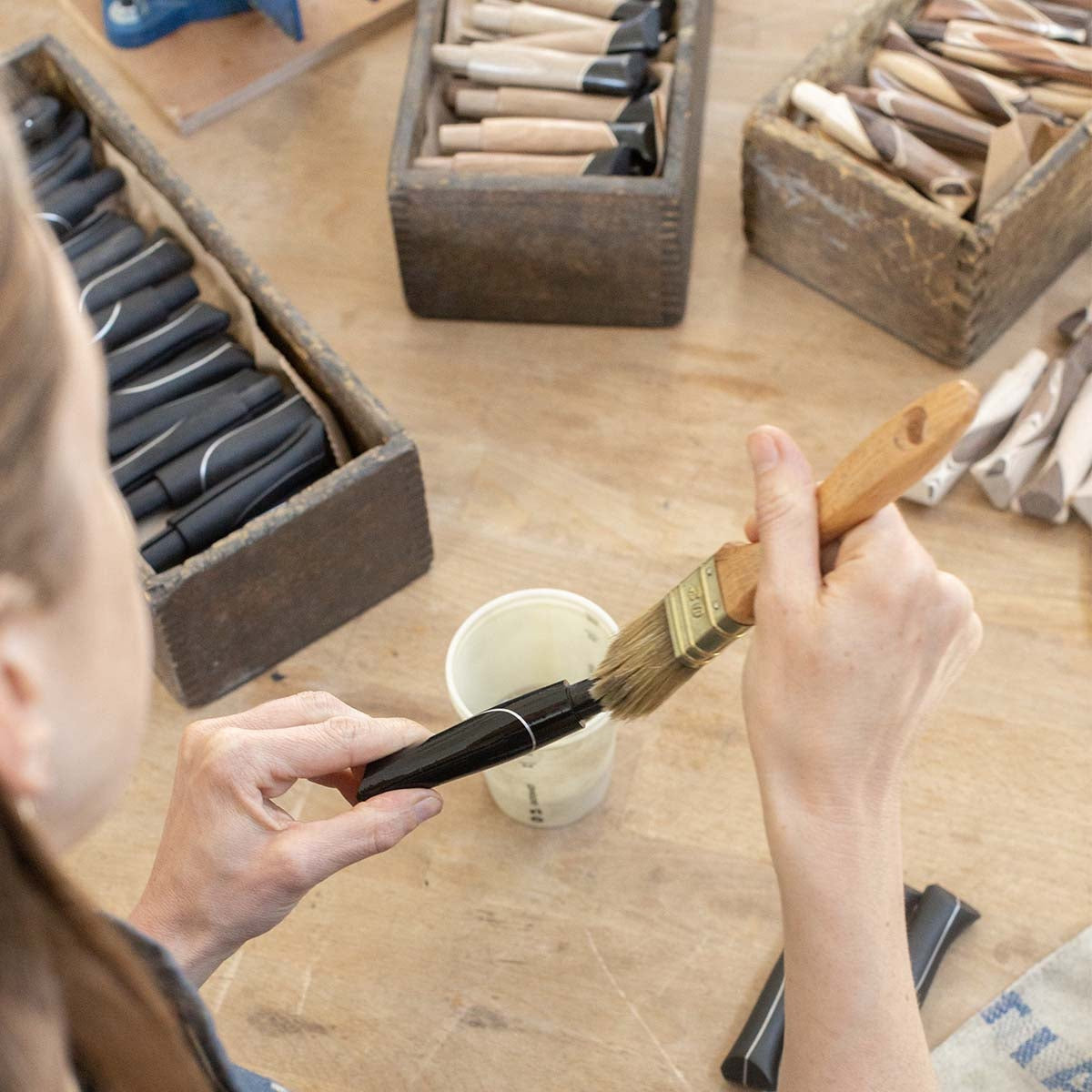In the photograph, a woman with light brown hair, partially visible from an over-the-shoulder angle, is meticulously painting a black, tubular object held tightly in her left hand. The paintbrush, gripped in her right hand, moves carefully across the object, suggesting she is applying a varnish or similar finish. Her right shoulder slightly obscures the camera's view, but her eye socket and earring are visible. The overall scene conveys a detailed painting process.

In front of her, an off-white plastic cup sits on a table, surrounded by three open boxes. These boxes contain a mix of similar objects in various stages of completion: some are entirely black, others are partially painted with black ends, and a few remain in their natural wood tones. One of the boxes, situated to the right, is filled with untouched materials. A cloth towel is also discernible at the bottom right-hand corner of the frame. The woman's aged hands, focused and steady, reveal her experienced touch as she works on the intricate hand-carved items that resemble whistles.